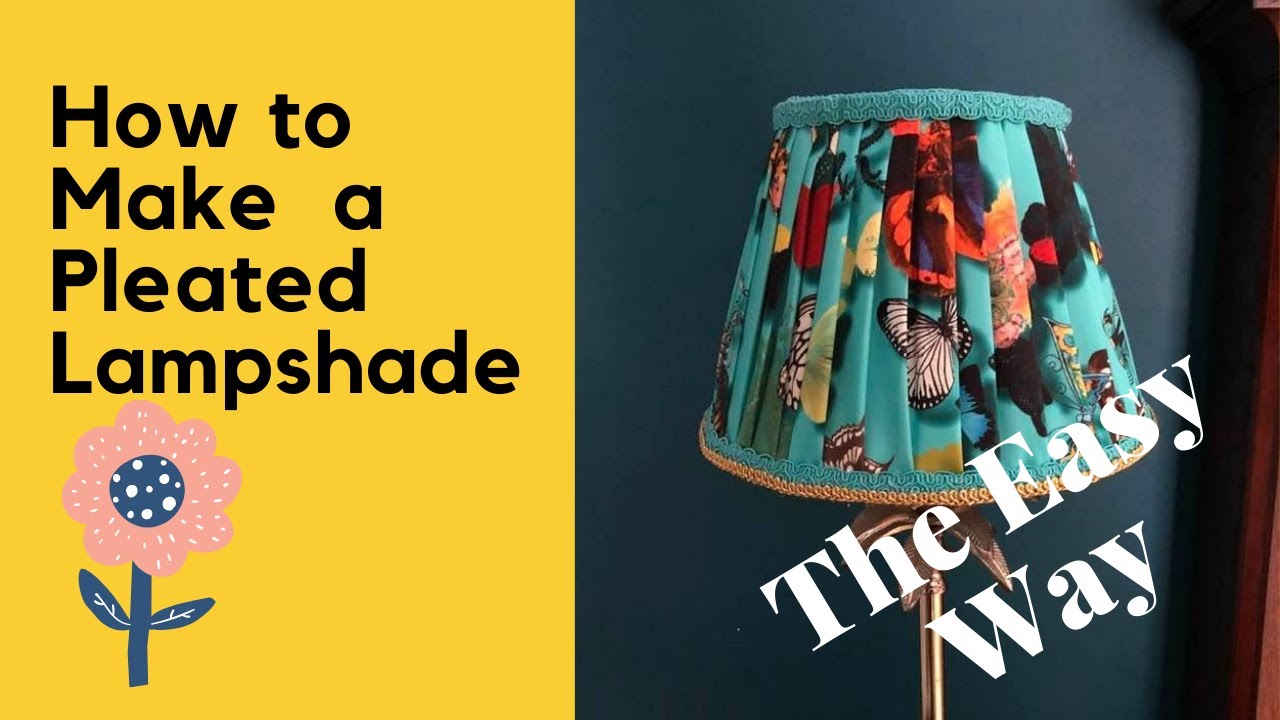This image resembles a Pinterest pin or a YouTube thumbnail, potentially for a DIY project or a website header. On the left, a section with a yellow background features black text that reads "How to Make a Pleated Lampshade," accompanied by a clipart of a pink and blue flower. On the right-hand side, there is a photo of a homemade pleated lampshade with a teal butterfly print, trimmed at the top and bottom. The lampshade, which is slightly tacky in appearance, is mounted on a tall, decorative gold floor lamp set against a navy blue wall. Finally, across the photo in white text are the words "The Easy Way."